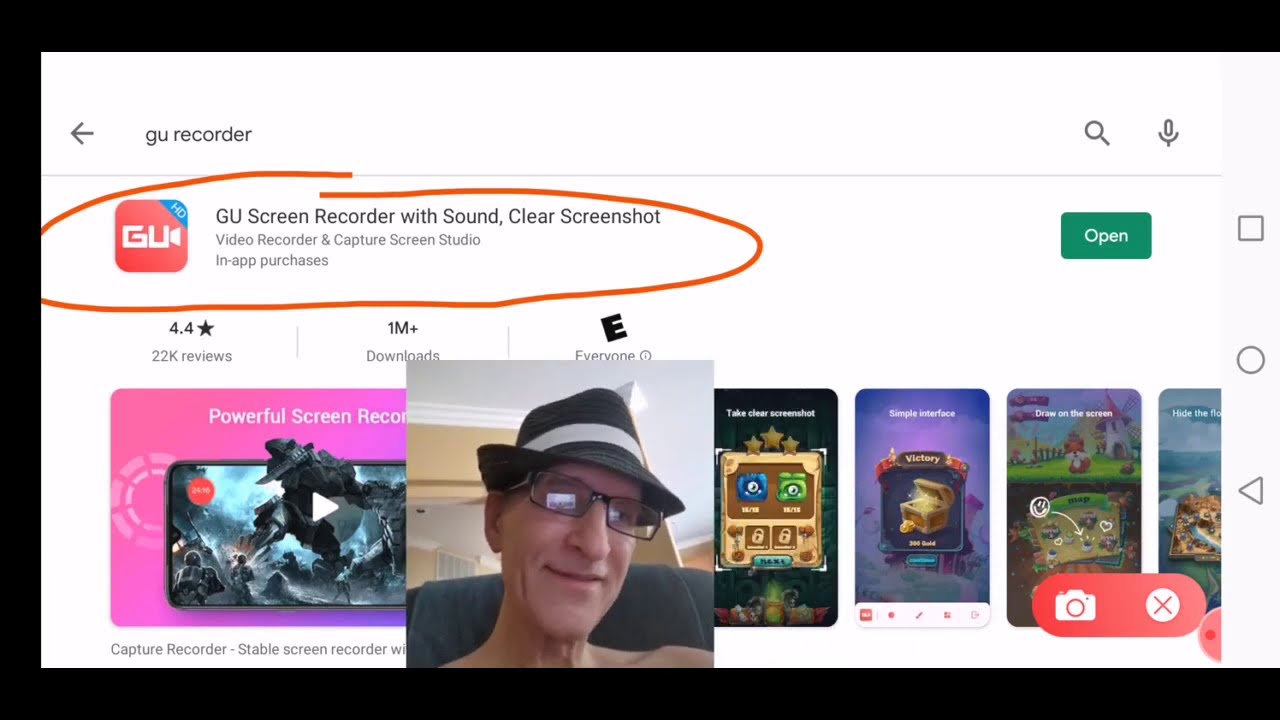This horizontal rectangular image is bordered by a thick black line on the top, bottom, and left edges, while the right edge is open for an unknown reason—possibly due to partial screen cut-off or the absence of a border. Within this border, set against a crisp white background, the top left corner features a left arrow followed by the text "GU recorder" in all lowercase letters. On the right, there are icons of a magnifying glass and a microphone.

A red oval encircles important content within the image. To the left of this circled area, there is an icon set against a red vertical rectangular background with the letters "GU" in white capital letters. Situated in the upper right corner of this rectangle, a small turquoise box with white text displays "HD" in capital letters.

The circled text reads, "GU screen recorder, clear screenshot." Beneath this, in a smaller font, it states, "Video recorder and capture screen studio," followed by, "in-app purchases." On the right side of the circled area, a green button with white text reads "Open."

Below this section, a series of images are present. The first image features a pink background with partially visible white text stating "powerful screen record." The image showcases a cell phone with a play button, indicating action or video playback. The second image, closer to the viewer, displays a man wearing glasses and a hat, seated on a sofa or chair.

Adjacent to these, a row of three and a half additional images is visible, although their details are harder to discern. Overlaying these images slightly is a horizontal red icon featuring a white camera on the left and a white X on the right.